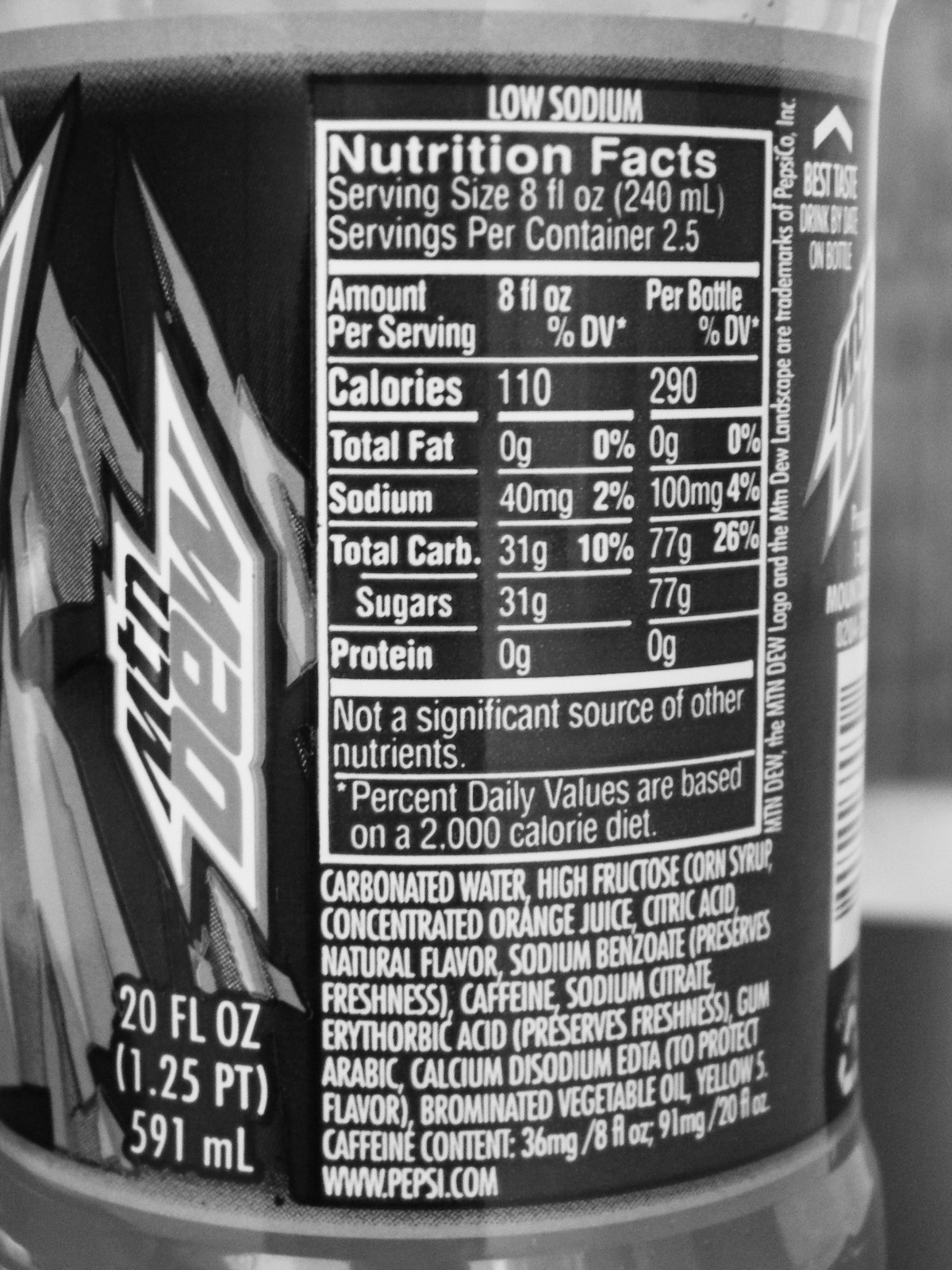This black and white photograph showcases a bottle of Mountain Dew prominently positioned against a plain backdrop. The recognizable Mountain Dew logo is displayed on the left side of the bottle. The label beneath the logo details the volume as 20 fluid ounces (1.25 pints, 591 milliliters). Notably, the bottle advertises "Low Sodium."

The nutrition facts provided on the label specify a serving size of 8 fluid ounces (240 milliliters), with the bottle containing approximately 2.5 servings. Each serving delivers:

- Calories: 110
- Total Fat: 0 grams
- Sodium: 40 milligrams
- Total Carbohydrates: 31 grams
- Sugars: 31 grams
- Protein: 0 grams

The label states that it is "Not a significant source of other nutrients" and notes that percent daily values are based on a 2,000-calorie diet.

The ingredients list details that the beverage contains carbonated water, high fructose corn syrup, concentrated orange juice, citric acid, natural flavor, sodium benzoate (to preserve freshness), caffeine, sodium citrate, erythorbic acid (to preserve freshness), gum arabic, calcium disodium EDTA (to protect flavor), brominated vegetable oil, and Yellow 5. The caffeine content is specified as 36 milligrams per 8 fluid ounces and 91 milligrams per 20 fluid ounces. The website www.pepsi.com is also listed on the label.